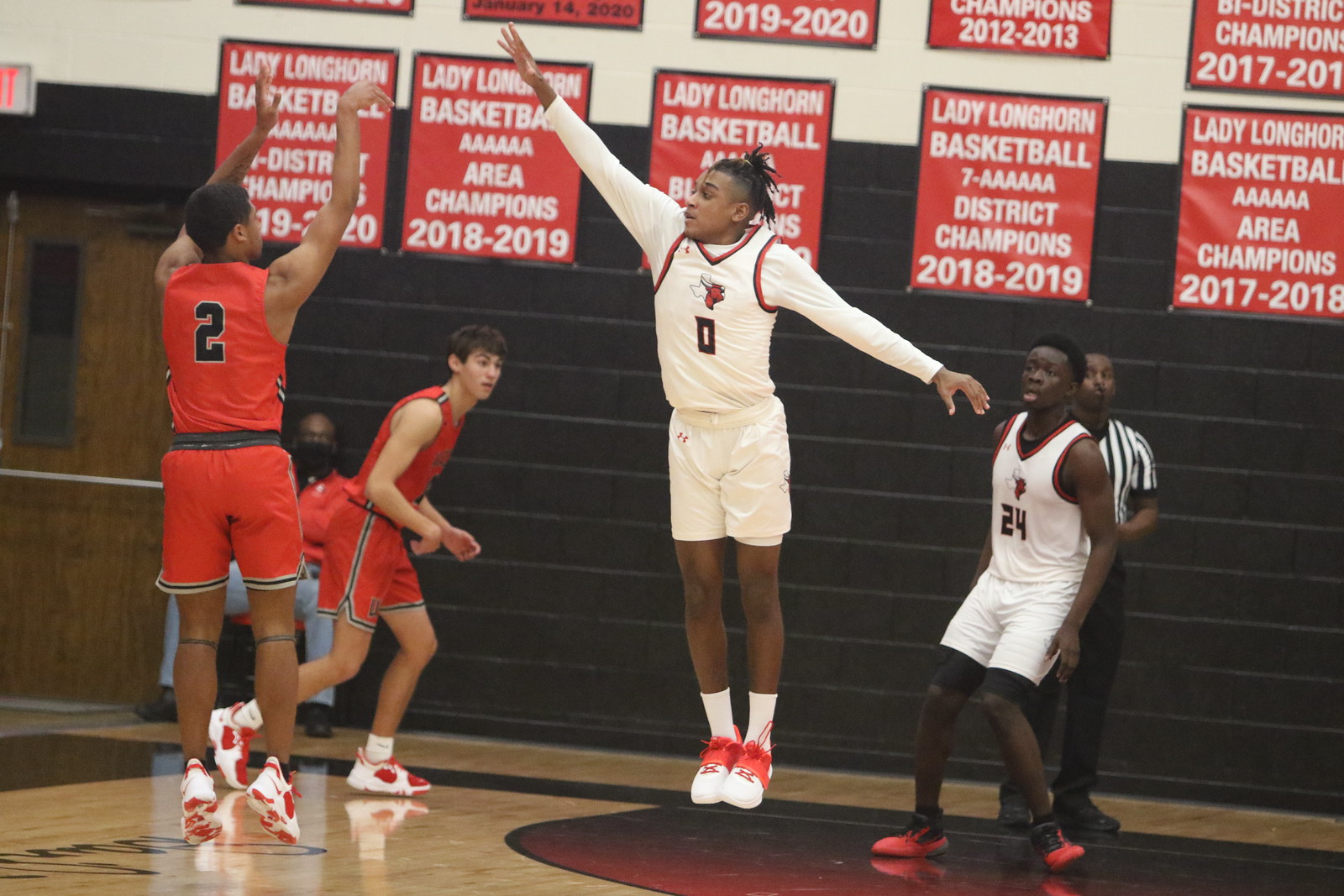This image captures a dynamic moment during a men's basketball game, likely at the college or high school level. Four players are prominently featured: two in white and two in red uniforms. At the center is a player in white, number 0, airborne with feet together and arms outstretched. Nearby, a player in red, number 2, is also in mid-air, demonstrating a follow-through pose after shooting the basketball. Another player in white, number 24, observes the action from the right-hand side. Behind them, a referee in a black and white striped shirt oversees the game, while a person in a facemask, red shirt, and jeans sits in the background. The gym's cinderblock wall is painted charcoal gray and adorned with numerous signs and plaques. Among them, posters with a red background and white lettering proclaim "Lady Longhorn Basketball" and document various championships such as "Area Champions 2018-2019." An emergency exit and a wooden door with a push bar can be seen on the left side of the image.